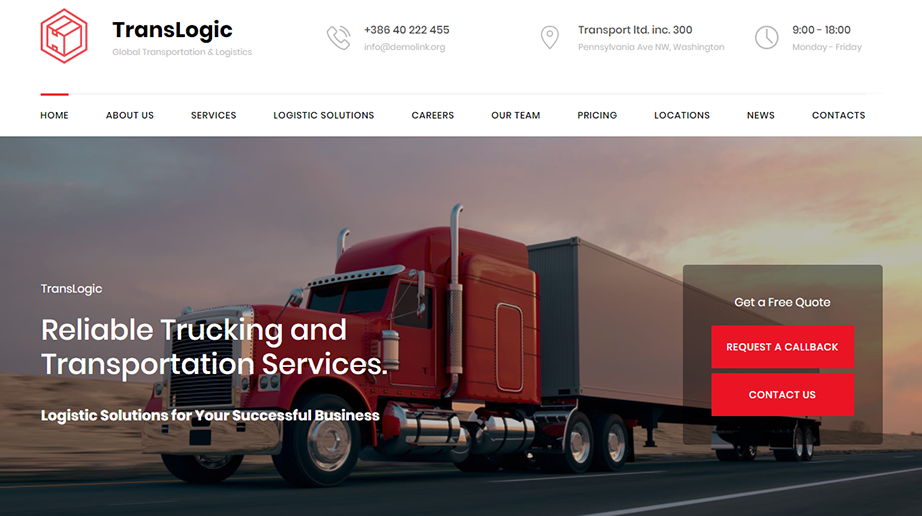**Caption:**

This image, intended for the website of Translogic—a global transportation and logistics company—features a striking visual of an 18-wheeler truck. The company name "Translogic" is prominently displayed in bold black text, accompanied by a distinctive red outline box. Below, contact information is provided, including a phone number (386-402-2455) and an email address accessible with low phone signal.

The company's address, "Transport Inc., 300 Pennsylvania Avenue, W Washington," and their operating hours (9:00 AM to 6:00 PM, Monday through Friday) are also listed. Navigation menu items such as Home, About Us, Services, Logistic Solutions, Careers, Our Team, Pricing, Location, News, and Contact are present.

The image depicts a meticulously maintained truck with a red front and a white trailer, traveling down an isolated highway under clear evening skies, resembling a desert landscape. The backdrop suggests a picturesque sunset. The truck and trailer don the name "Translogic" in white, underscoring the caption "Reliable trucking and transportation services. Logistics solutions for your successful business."

Additional elements include a black box with "Get a free quote," and red boxes for "Request a call back" and "Contact us," all in white text, making it easy for potential clients to take immediate action.